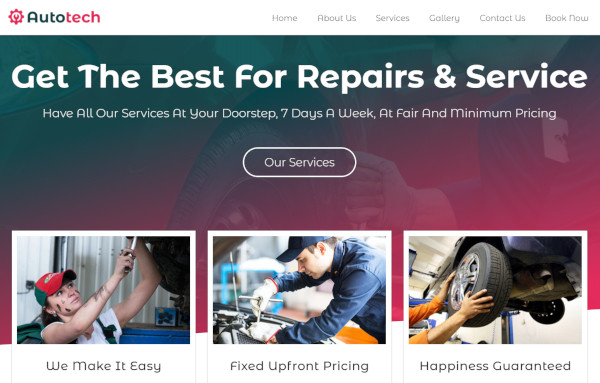The website features a predominantly black-to-red gradient background with a bold and modern aesthetic. At the top, the logo stands out with "Auto" written in dark gray or black and "Tech" in a vibrant pinkish-red. Navigation links across the top menu include: Home, About Us, Services, Gallery (though misspelled), Contact Us, and Book Now.

In the central banner, a prominent white slogan declares, "Get the best for repairs and service." Just below, in smaller gray text, a secondary message promises, "Have all our services at your doorstep, seven days a week, at fair and minimum pricing." There is also a call to action button inviting users to "See Our Services."

Below the banner, the website showcases three images of mechanics working on cars. The first image features a lady reaching up to work on a car elevated on a rack with the caption "We make it easy." The second image shows a man leaning over a car with the phrase "Fixed up front by pricing." The final image depicts a person attempting to remove a tire, accompanied by the assurance "Happiness guaranteed."